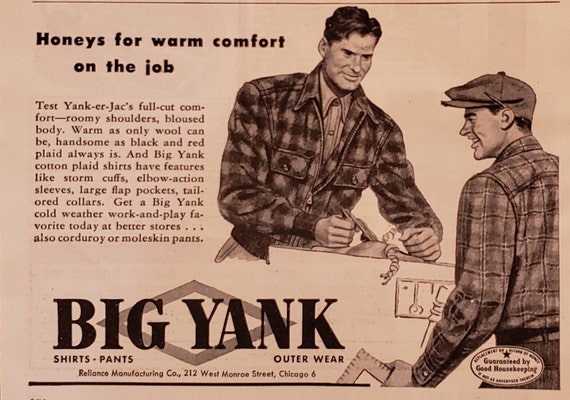This image is an advertisement for Big Yank, featuring their line of shirts, pants, and outerwear. The ad has a pinkish or brownish background, resembling scanned paper. Prominently displayed on the top left is the slogan, "Honeys for warm comfort on the job," in bold, black letters. Below the slogan, a detailed paragraph describes the clothing line, highlighting features like storm cuffs, elbow-action sleeves, and large flat pockets.

On the right side of the ad are two graphic images of men wearing plaid shirts. One man, with glossy black hair and a collared undershirt, is depicted working on something in front of him. The other man, wearing a 1930s style hat and a grayish striped shirt, holds a triangular ruler and gazes at the text.

At the bottom left corner, the Big Yank logo is prominently displayed with bold, black letters over a dull, sideways diamond shape. The text underneath reads, "Big Yank Shirts, Pants, Outerwear," followed by the address: "Reliance Manufacturing Co., 292 West Monroe Street, Chicago 6." A small oval in the bottom right corner indicates that the ad is sponsored by Good Housekeeping.